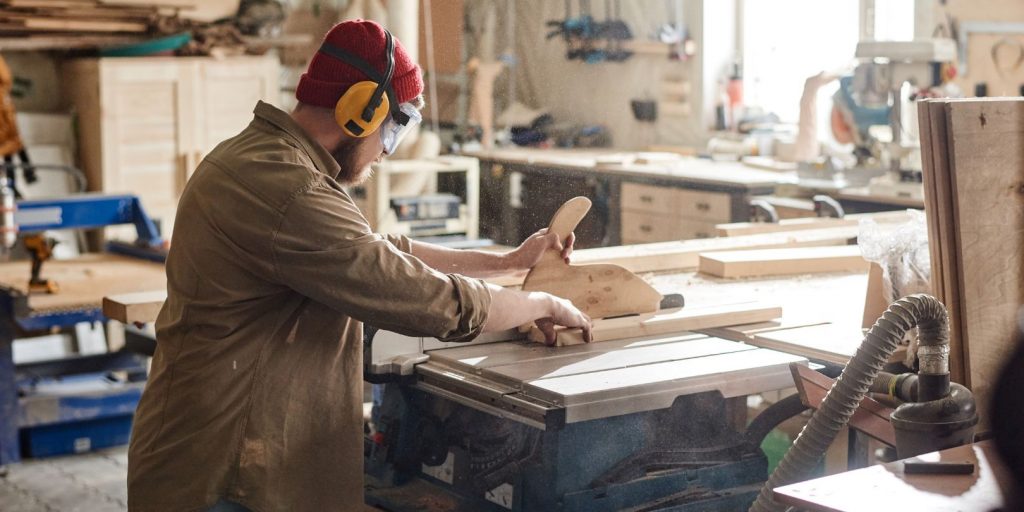A worker dressed in brown long-sleeve attire, with the sleeves rolled up to just below his elbows, is engrossed in cutting wood in a workshop. He wears yellow ear protection headphones with a black connecting band, enhancing his safety along with a red hat perched on his head. Clear safety goggles with black straps secure around his head, shielding his eyes as he meticulously cuts a block of wood on a wooden work surface. His left hand grips a wood-colored cutter, showcasing his focus and precision as he works in this detailed, safety-conscious setting.